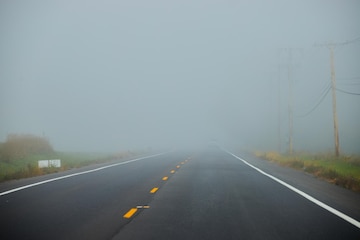This image depicts a forlorn-looking, newly paved highway disappearing into a dense fog that obscures the distant horizon. The road is a two-lane, slate-gray stretch of smooth asphalt with freshly painted markings: vibrant yellowish-neon dashed lines in the center and crisp white lines on the edges. Sparse vegetation, including grass and shrubs, grows alongside a narrow shoulder, suggesting a rural or semi-rural setting. Dilapidated wooden telephone poles with sagging cables line the right side of the road, gradually vanishing into the fog. On the left, near a small mound or hill, stands a white sign. The fog shrouds much of the scene, creating a bleak, desolate atmosphere.